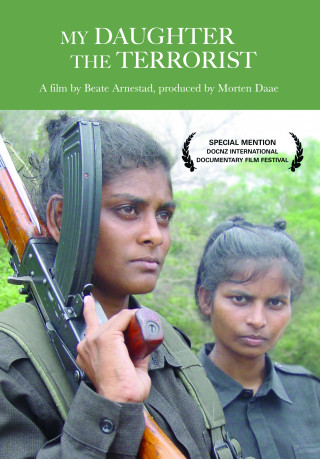The poster depicts an advertisement for the film "My Daughter the Terrorist," directed by Beat Orensted and produced by Morton Day. The image showcases two South Asian women dressed in military-style uniforms, standing amidst a forest. The woman on the left, who appears to be younger, has brown skin and black wiry hair, and is wearing a green vest over a dark charcoal collared shirt. She is holding a rifle with a brown wooden stock and a black metal component, looking to the right. The woman on the right has similar dark hair, is also wearing a collared shirt, and is staring directly at the camera. Above the image, set against a green background, the film's title is prominently displayed in white text. To the right of the image, there is additional text in black, surrounded by laurel designs, that reads "Special Mention DOCNZ International Documentary Film Festival," recognizing the film's accolade.